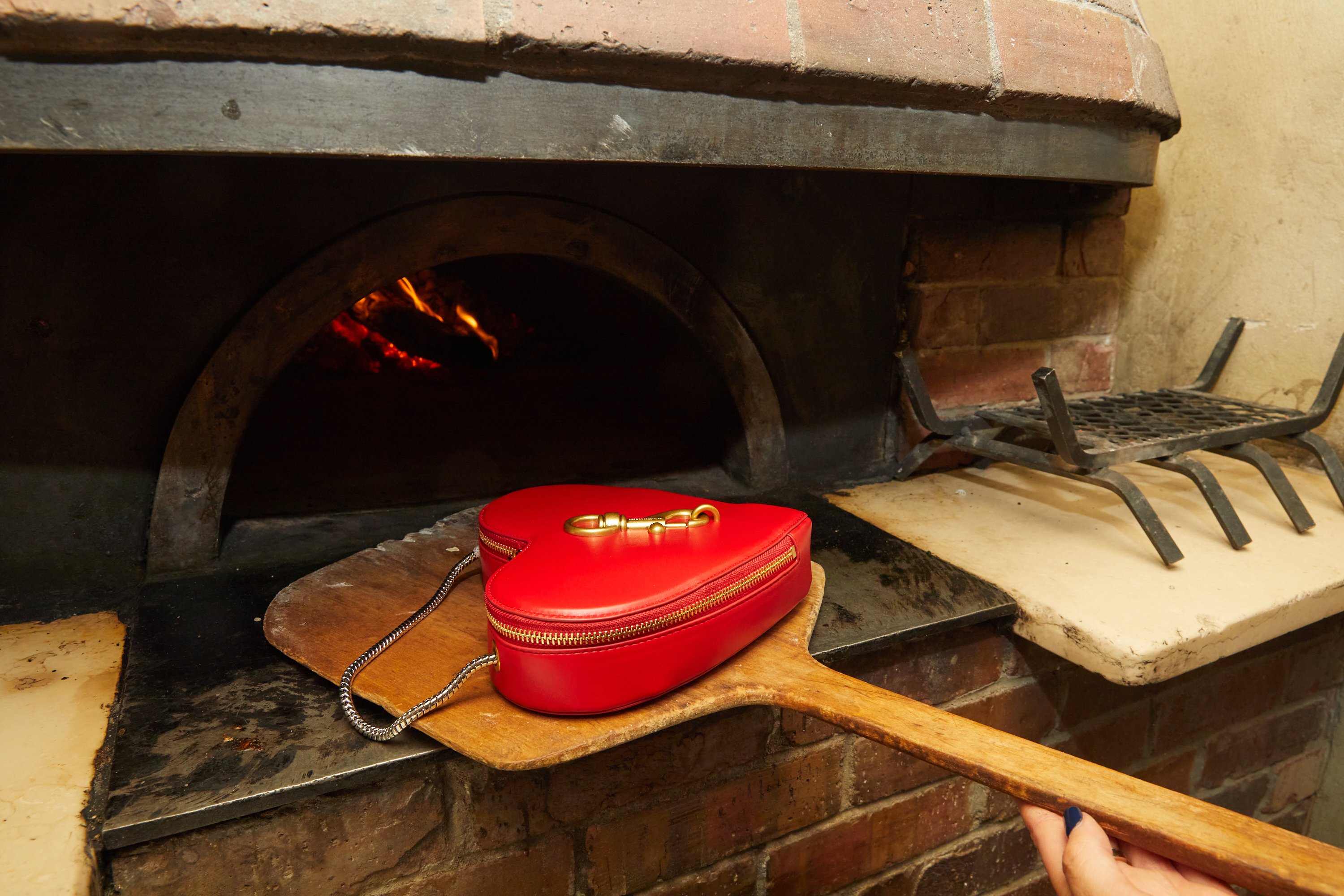This photograph captures a rustic, old-style pizza oven, predominantly constructed from red bricks and featuring a half-moon shaped opening. The central section of the oven includes dark, almost black metal, around the opening, and there is visible fire burning inside. To the oven’s right, there is a metal rack sitting on a concrete slab, likely used for cooking preparations. On the left, a small concrete area is partly visible.

A wooden pizza paddle, originating from the bottom right corner of the image, extends towards and into the middle of the frame, held by a female with blue fingernails on her left hand. Instead of a pizza, this paddle supports a conspicuous, heart-shaped red purse. The purse is glossy, with a golden metal attachment at the center, a silver chain handle, and gold-colored zipper detailing. The juxtaposition of the burning oven and the delicate purse creates an intriguing and whimsical scene, indicative of a playful, imaginative context.